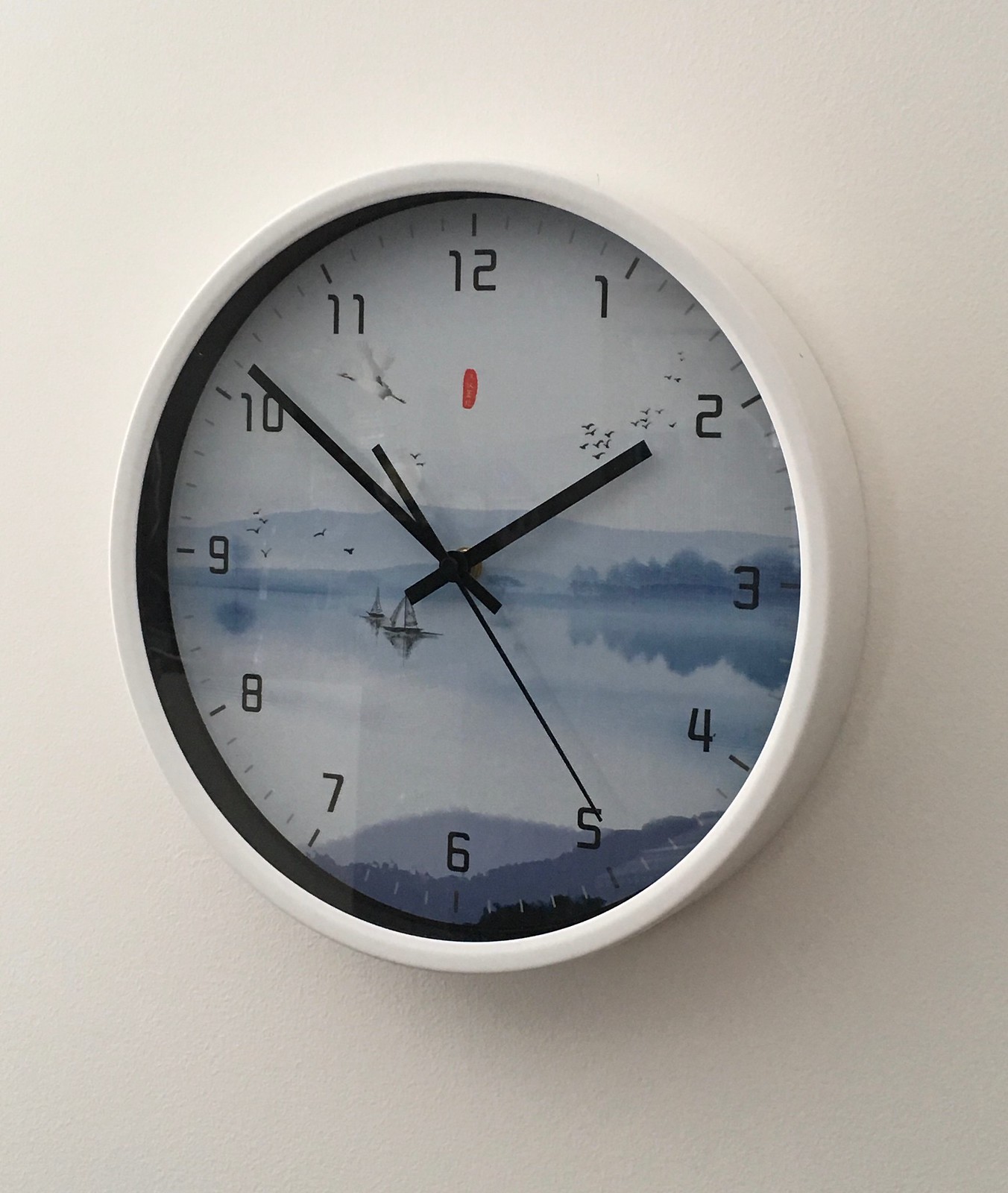This image features a round white clock hanging on an off-white, subtly textured wall. The clock has a clean, white bezel frame and black hands, including a long, thin second hand. The inside of the clock isn’t a typical face with numbers; instead, it showcases a serene landscape scene. The backdrop within the clock depicts a light gray and blue nature setting, including distant grayish mountains and foothills, light gray trees on the right, and a bluish waterway in the center. In the foreground, there are some bushes and shrubbery, while a pair of small sailboats glides on the reflective lake. The sky is decorated with birds and ducks, adding to the tranquil scenery. The clock hands point to 2:11, with the hour hand slightly past 2, the minute hand just past 10, and the second hand on the 5. The clock runs from 12 at the top, going around back to 12 again, featuring a modern, computer-like font for the numbers.